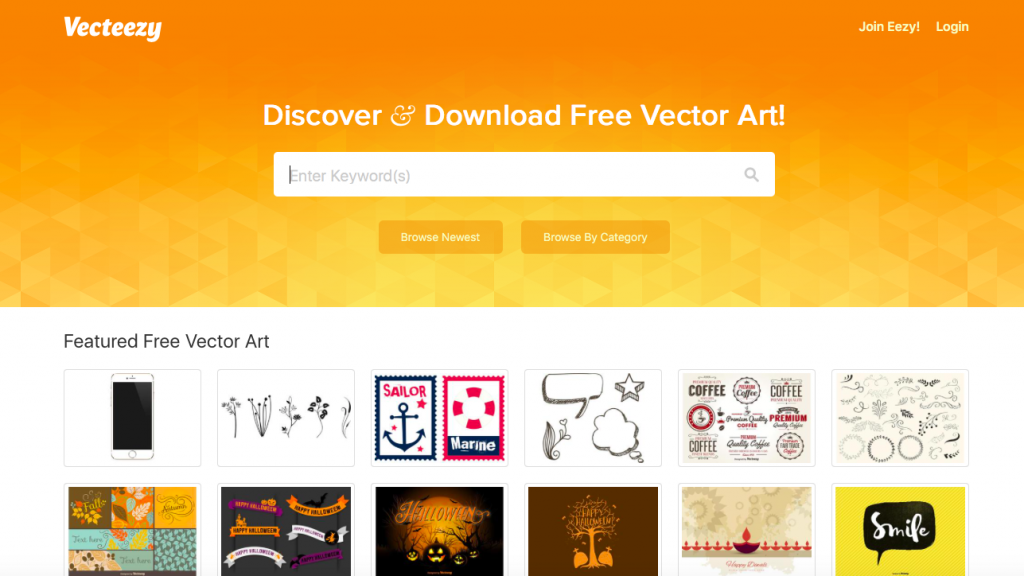This image appears to be a screenshot from a website, likely showcasing a platform for downloading vector art. The top portion features a prominent orange rectangle that blends into yellow at the bottom, adorned with a subtle cube pattern, creating an ombre effect. In the upper left corner, "VectEasy" is displayed in white font, while the options to "Join" and "Log In" are situated on the upper right.

Central to the image, in white text, are the words: "Discover and download free vector art." Directly below this is a search bar with the placeholder text "Enter keywords," accompanied by a search icon. There are also options to "Browse newest" and "Browse by category" listed underneath.

The background shifts to white further down, where black text on the left reads: "Theatre to free vector art." A variety of vector art samples are displayed across this section. These include an illustration of a mobile phone in black, a black-and-white drawing of flowers, an anchor on a stamp, various speech or thought bubbles, and circular stickers. Additional artwork includes round designs on a cream background, multi-colored circles at the bottom, wavy lines and curves, an image resembling a cave with monster eyes peeking out, an orange tree, a close-up of a shell in grey and beige tones, and a piece with a yellow background featuring a black speech bubble containing small white text.